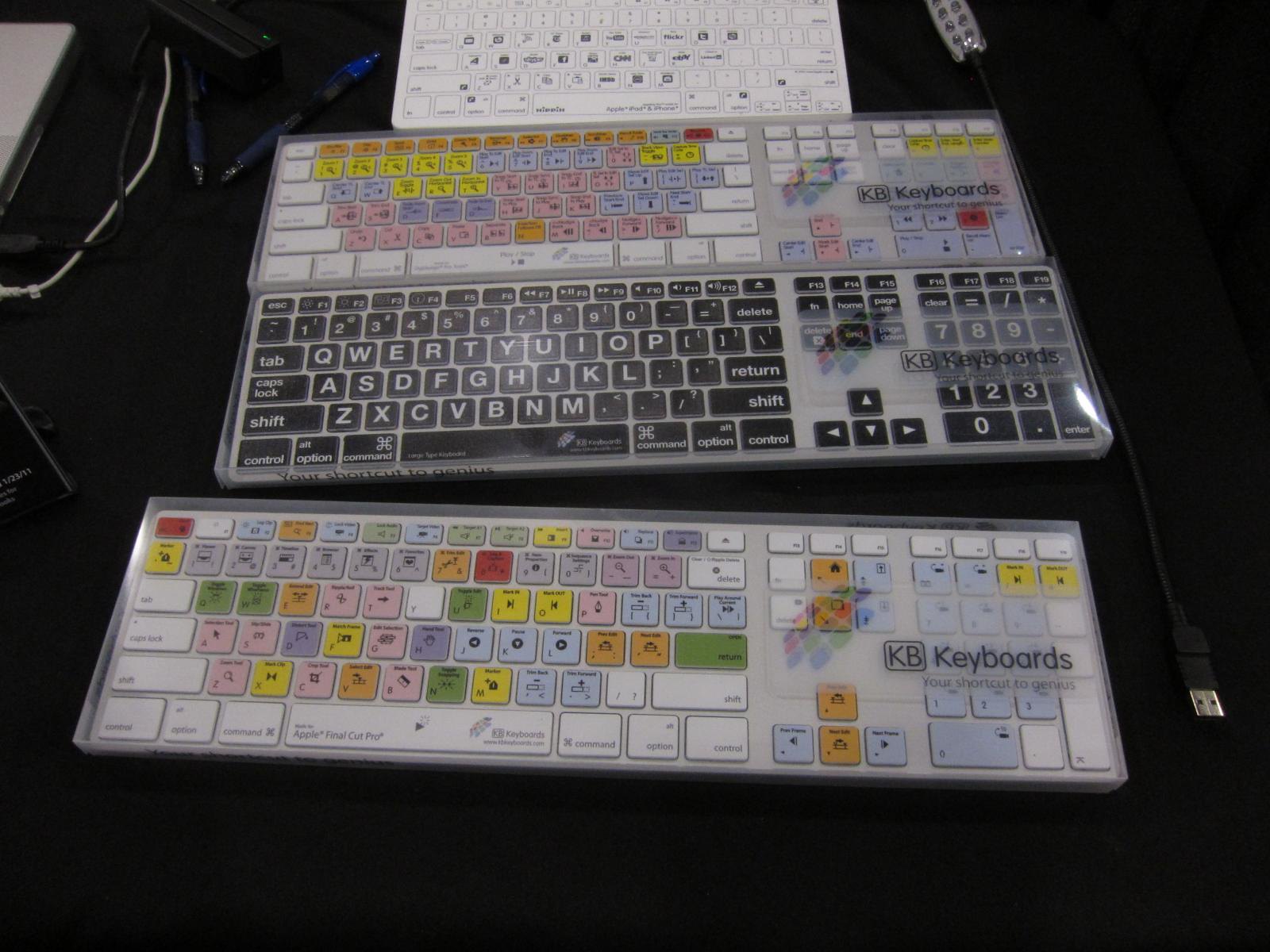The image depicts a dark, almost black, background featuring an array of keyboards and various electronic accessories. In the upper left corner, a few USB cables and electronic devices, as well as two ballpoint pens—one with a blue click-top and another indistinguishable—can be seen. A cord runs down the right side, likely for a phone or computer. Centrally, there are four keyboards. At the top, a white keyboard with dark characters on its keys appears too small to discern specific details. Below it sits a colorful, non-ergonomic rectangular keyboard branded with "KB Keyboards," protected by a clear plastic cover. This keyboard is adorned with a vibrant mix of green, pink, orange, yellow, red, purple, and lavender keys arranged in a meticulous color-coded pattern. The third keyboard from the top is designed for low-vision users, featuring large white letters on black keys, and is also marked with "KB Keyboards". Finally, the bottom keyboard mirrors the colorful KB design, sporting a different but equally vivid array of gray, white, yellow, orange, red, pink, purple, and green keys, similarly shielded by a plastic cover.